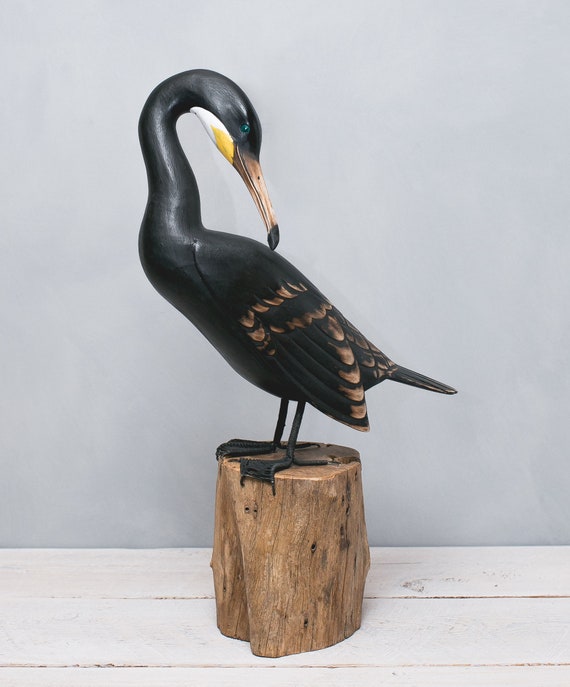The image depicts a painted sculpture of a tall, black bird standing on a wooden log placed on a white plank floor against a gray background. The bird, which resembles a black mallard, has a glossy black body with beige-tipped feathers on its wings and tail. It has a long, curved neck that forms a question mark shape as it extends upward and then bends downward. The beak is primarily beige with a darkened base and black tip, and there are yellow and white feathers underneath the chin. The bird has striking green eyes and stands on long, skinny legs with webbed feet, suggesting a meticulous level of craftsmanship in this custom-made sculpture.